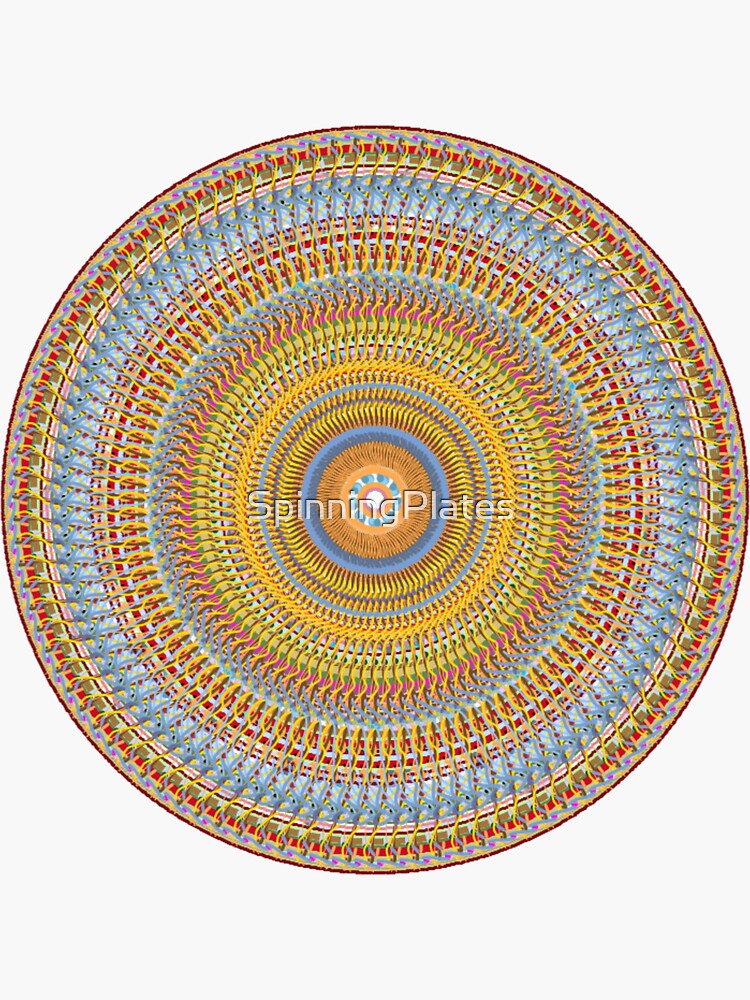The image depicts a vibrant and intricate piece of digital art resembling a mandala or an elaborate woven rug, set against a light gray background. This large circular design features a complex repeating pattern of concentric rings, each ring showcasing a diverse array of colors including purples, blues, reds, yellows, pinks, greens, oranges, and violets. As the pattern radiates outward from the small off-white center, the hues transition through various shades, creating a mesmerizing gradient effect. The intricate design appears almost tangible, reminiscent of finely woven fabric or a beautifully decorated plate. Central to the piece is a watermark reading "spinning plates," subtly blending into the detailed artistry. The outermost edge of the pattern is marked by a thin, dark brown rim, encapsulating the vibrant spectrum within.